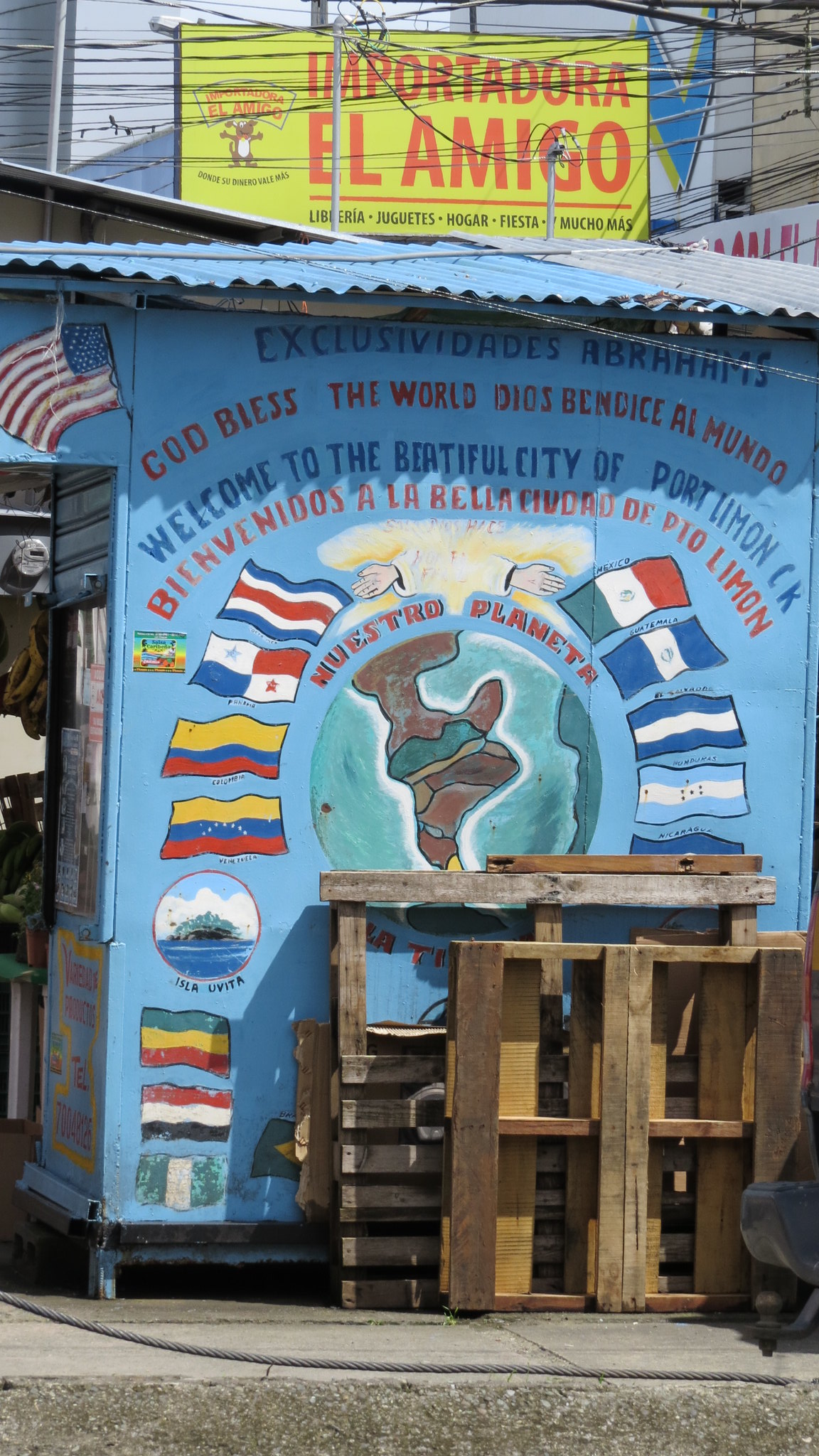This is a color photograph of the front of a blue-painted building, likely a business in Mexico. Prominently displayed at the top is a yellow sign with red text that reads “Import Adora El Amigo.” Below the sign, a blue corrugated metal awning shades portions of the building. The façade of the building is predominantly light blue with various text and imagery. In a darker blue font, the building features text that includes "Exclusivitis" and "Excluidas Eberharms." Additionally, the phrases "God Bless the World" and "Welcome to the beautiful city of Port Limon Sique Bienvenida Nuestro Planeta" are written, mixing both English and Spanish languages. 

The mural on the wall beneath the text includes a colorful depiction of a globe, highlighting Africa with aquamarine oceans. Around this globe, there are numerous flags representing different countries—14 in total, though some are partially obscured by three wooden pallets in front of the wall. The area in front of the building includes a sidewalk and a patch of grass. Overall, the image is vibrant with rich details showcasing a multicultural theme.